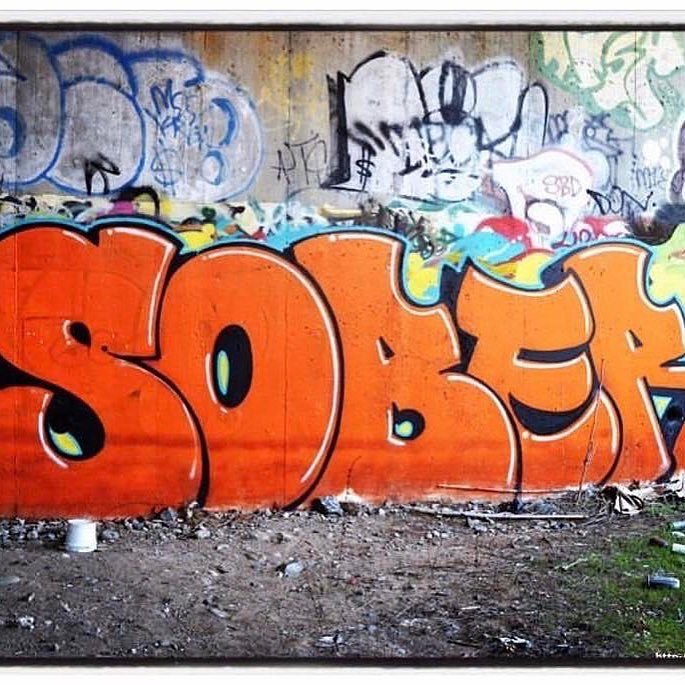The image depicts a concrete wall adorned with various forms of graffiti, most prominently featuring the word "S-O-B-E-R" written in large, bold, reddish-orange letters outlined in black and white. This striking piece of graffiti dominates the lower portion of the wall. Above it, the wall is cluttered with older graffiti, comprised of white circles with blue borders, black and blue spray-painted gang tags, and miscellaneous writing, including tags that read "S-B-D," "DAWN," and "W-S-U" in green and white. The scene appears to be situated in a dark, tunnel-like area or possibly beneath a bridge, as suggested by the shadowy ambiance. The ground below is a mix of dirt, rocks, trash, and some greenery, with a white, upside-down bucket on the left side adding to the sense of neglect and decay.